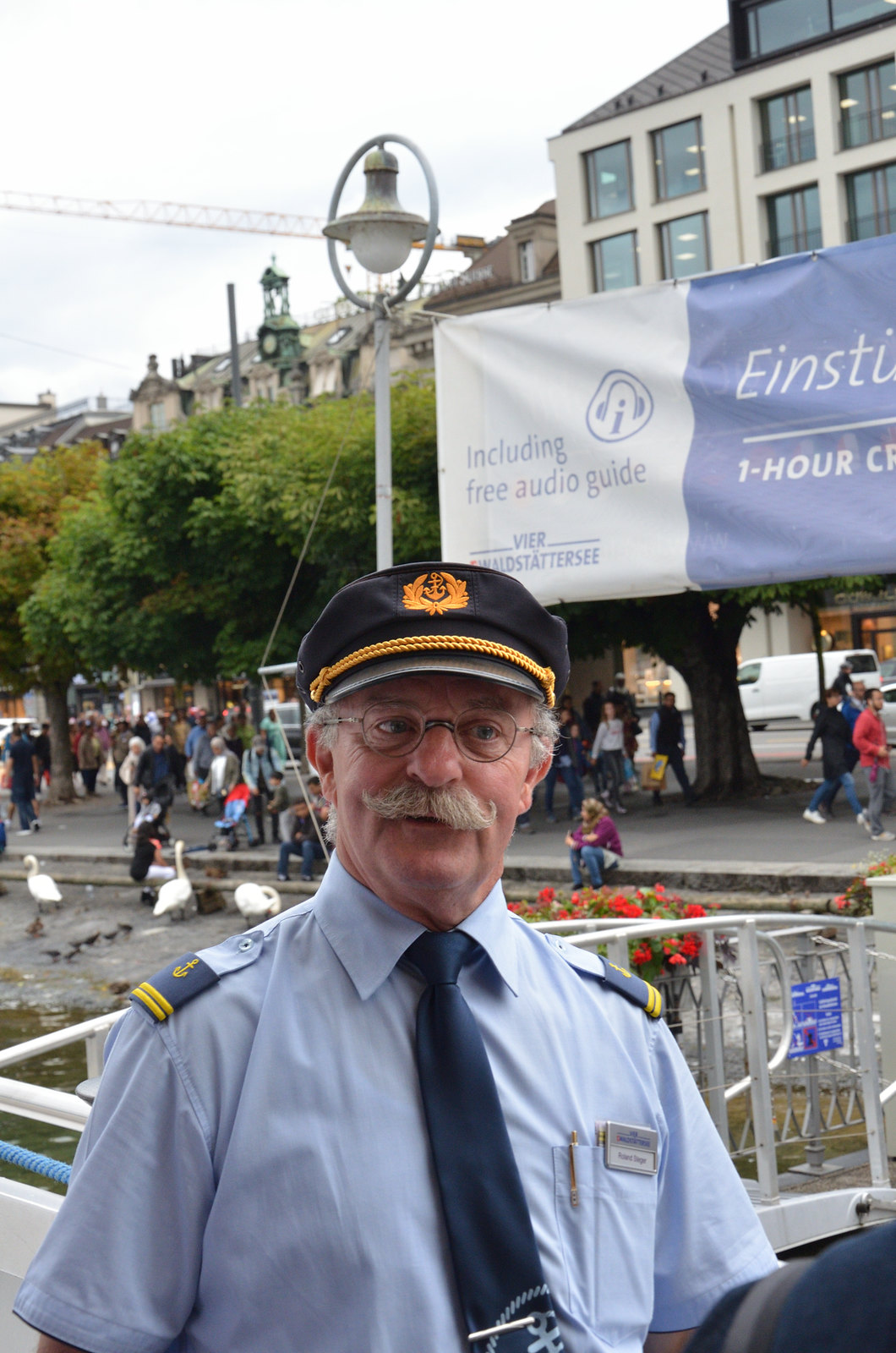An older man, dressed in a sea captain's uniform, stands in front of a scenic backdrop. His ensemble features a navy blue captain's hat adorned with gold embroidery and a gold emblem at the top, paired with a light blue short-sleeved shirt that has dark blue epaulettes with anchors and a matching dark blue tie. He sports round glasses, a thick curled gray mustache, and gray hair. A silver clip secures his tie, and a name tag is pinned to his shirt. Behind him, we see a fence leading to a greenish waterway with a few geese and other birds swimming. A cobblestone walkway with people strolling along it stretches out in the background, flanked by trees with green leaves and brown trunks. Among the structures visible, there are buildings with varied architecture—some with tan sides, others with brown and black roofs, as well as a white van and some other cars parked nearby. The sky appears white, and a blue sign hangs in the background along with a banner that reads "including free audio guide." Adding to the picturesque scene are red flowers, several steps where people are seated, and a construction crane peeking from behind the trees.